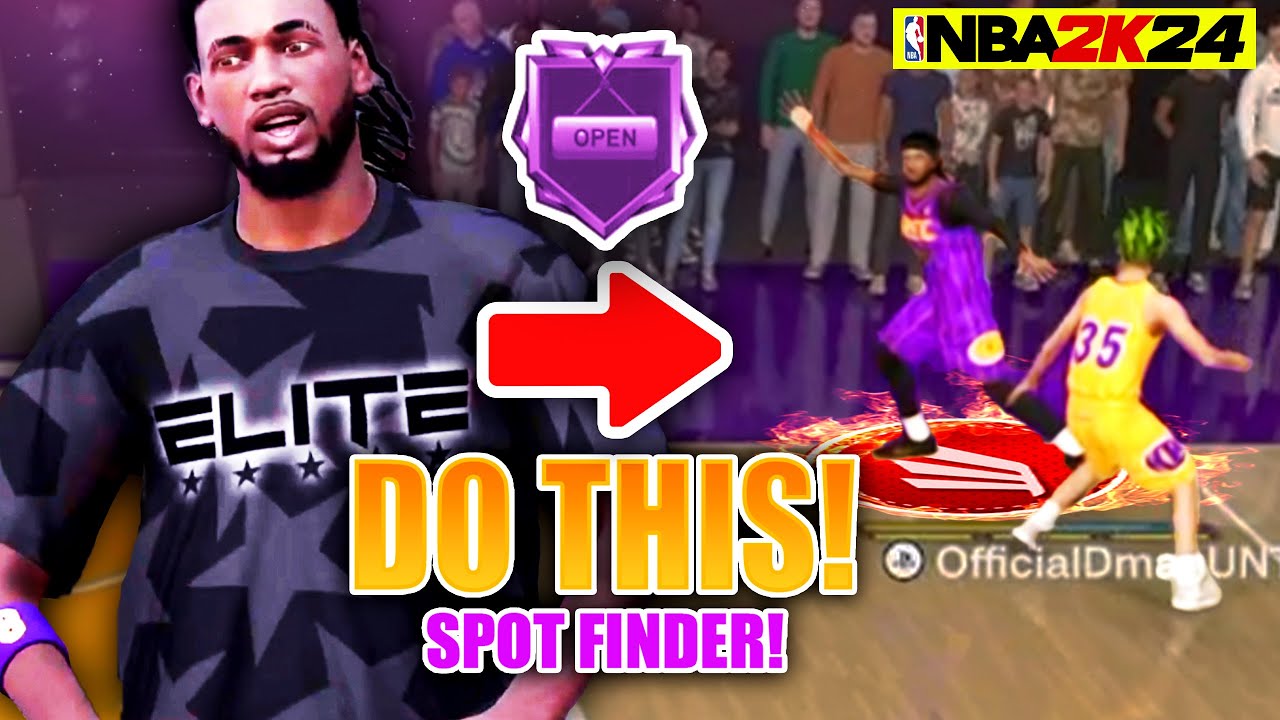This is an image from the animated video game NBA 2K24. The screenshot showcases a basketball-themed scene featuring an African American male character wearing a shirt with the word "ELITE" printed on it. The game's animated style is vividly displayed, and the scene is set on a detailed basketball court. Two teams are visible, one dressed in gold and purple, while the other team is adorned in purple and gold.

The court is surrounded by enthusiastic fans standing right on the sidelines, adding an extra layer of immersion to the game. A standout player in gold is notable for his unusual green hairdo, contributing to the vibrant and diverse character designs typical of the game.

Additionally, there's a prominent interface element labeled "Spot Finder" with text suggesting it is part of an in-game feature, displaying "Official D.M.A. Unit" which may relate to gameplay mechanics. Although there are no players dribbling the ball in this particular frame, the presence of the NBA branding firmly indicates that the game is basketball-focused.